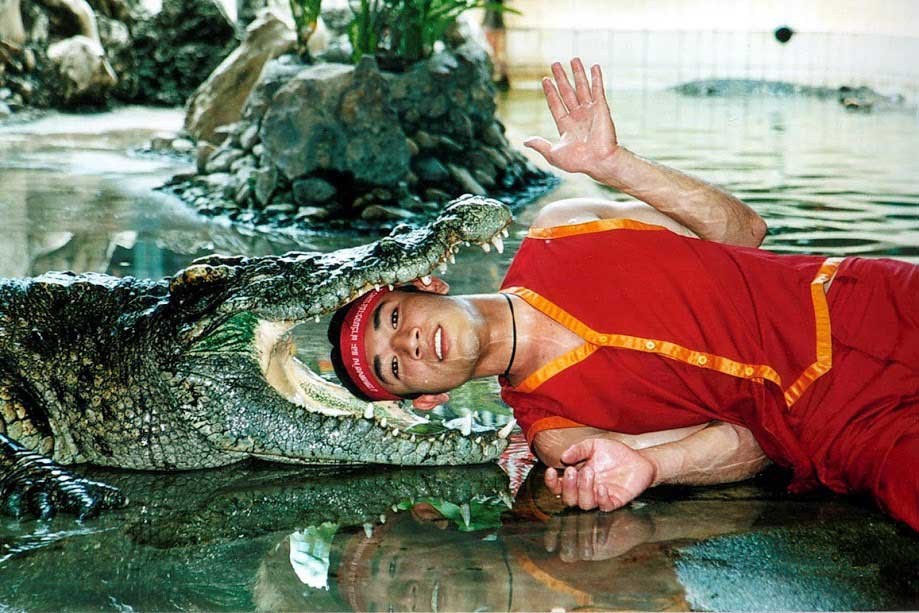In this intriguing and slightly unnerving image, a young man dressed in a vibrant red suit with orange trim is seen interacting with a crocodile in what appears to be a man-made sanctuary. The setting resembles an indoor park designed to look like the outdoors, with water flanking both the left and right sides. On the left side of the image, rocky terrain and a portion of a fence are visible, contributing to the naturalistic scene.

The crocodile, characterized by its green and brown scales marked with black spots, has its mouth wide open, revealing large, pointy teeth. Positioned towards the right, the crocodile's head and part of one foot dominate the left side of the frame. The young man, who might be Thai, wears a distinctive red headband with white Thai writing and is laying his head inside the crocodile's mouth, which creates a dramatic focal point at the center of the photograph. The man's daring pose and the ominous positioning of the crocodile enhance the overall tension and wildness of the scene.